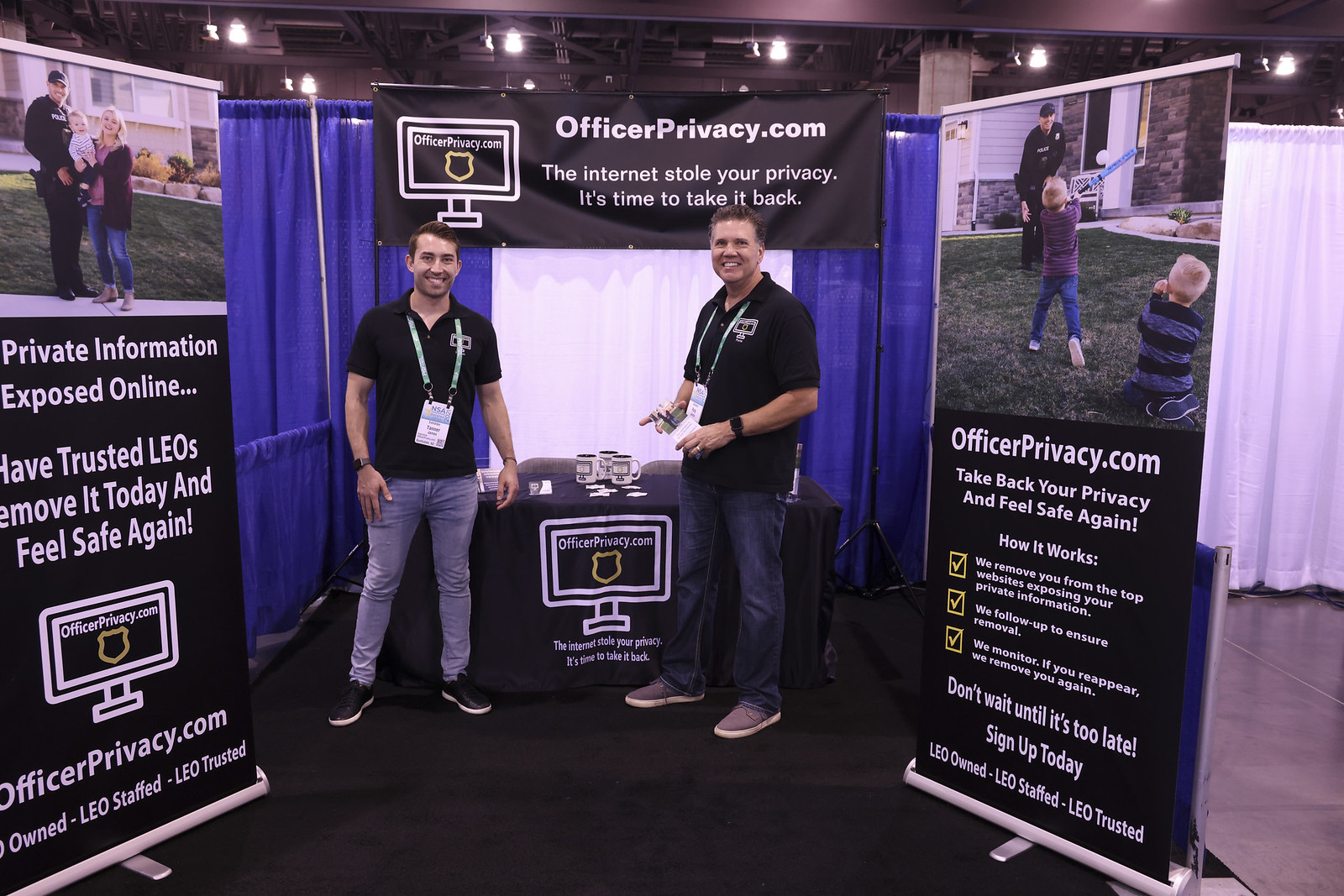The image is a detailed photograph taken at a conference booth for OfficerPrivacy.com. Central to the image are two men dressed in black shirts and blue jeans, both wearing green lanyards. They are positioned in front of a table draped with a black tablecloth, which prominently displays the text, "OfficerPrivacy.com, the Internet stole your privacy. It's time to take it back." Above them is a black banner featuring a graphic of a black desktop with a white monitor and the outline of a gold badge, reiterating the same privacy message.

Surrounding the duo are three standing banners. To the left, a sign reads, "Private information exposed online? Have trusted LEOs remove it today and feel safe again. OfficerPrivacy.com." Off to the right, another sign instructs viewers, "OfficerPrivacy.com, take back your privacy and feel safe again. How it works: Don’t wait until it’s too late, sign up today." This sign likely includes smaller text with further details, harder to discern, which also includes images of a family and children playing.

Behind the men is a curtained-off area, adding to the booth's setup. The two men appear engaged, perhaps smiling and pointing at their setup or computer, creating an inviting atmosphere for conference attendees.

This composition effectively emphasizes the privacy services provided by OfficerPrivacy.com, ensuring a clear and persuasive message to onlookers.